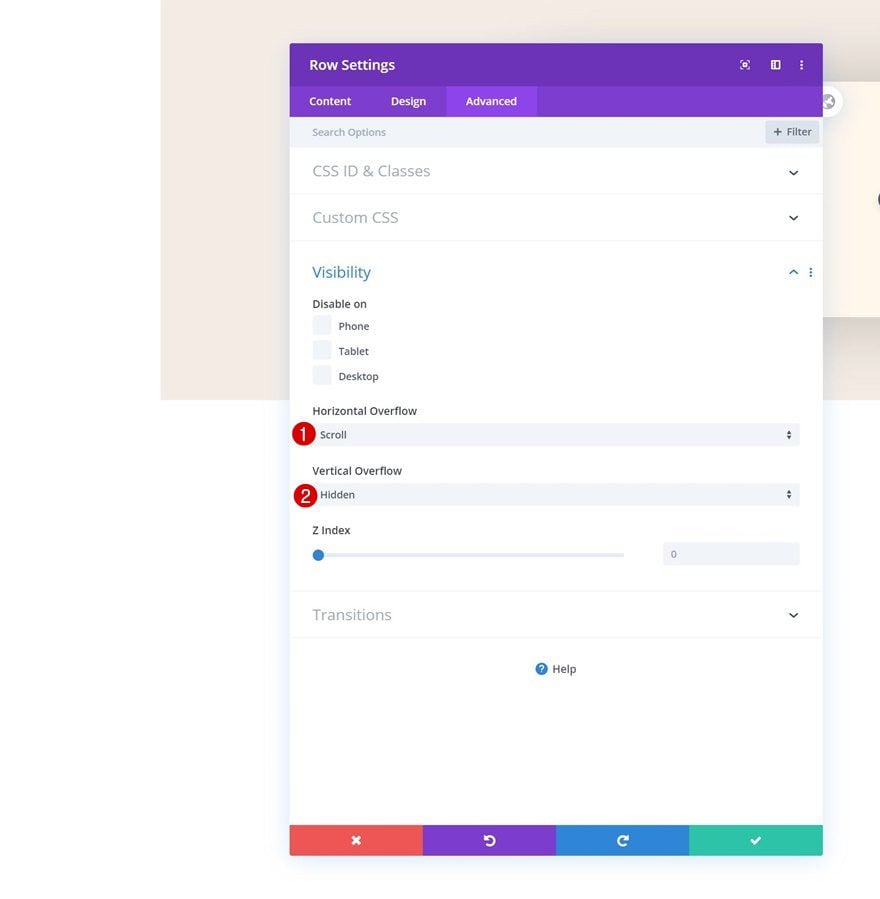The image is a screenshot of a web application interface, specifically within a settings page. In the top left corner, the title "Row Settings" is prominently displayed. Below the title, there are three tab options arranged horizontally: "Content" on the left, "Design" in the middle, and "Advanced" on the right. The "Advanced" tab is slightly highlighted, indicating that it is the active selection.

The main body of the page features a search bar at the top. Directly beneath the search bar are clickable links, with labels such as "CSS ID & Classes" and "Custom CSS." The interface is segmented into two distinct sections, each clearly marked by red circles containing the numbers '1' and '2'.

Section number one, denoted by a red circle labeled '1,' is titled "Horizontal Overflow." This section contains a toggle bar set to "Scroll." Immediately below it is section number two, identified by a red circle labeled '2,' titled "Vertical Overflow." This section features a toggle bar set to "Hidden."

The detailed layout and highlighted elements suggest a focus on advanced customization options, particularly for managing content overflow both horizontally and vertically.